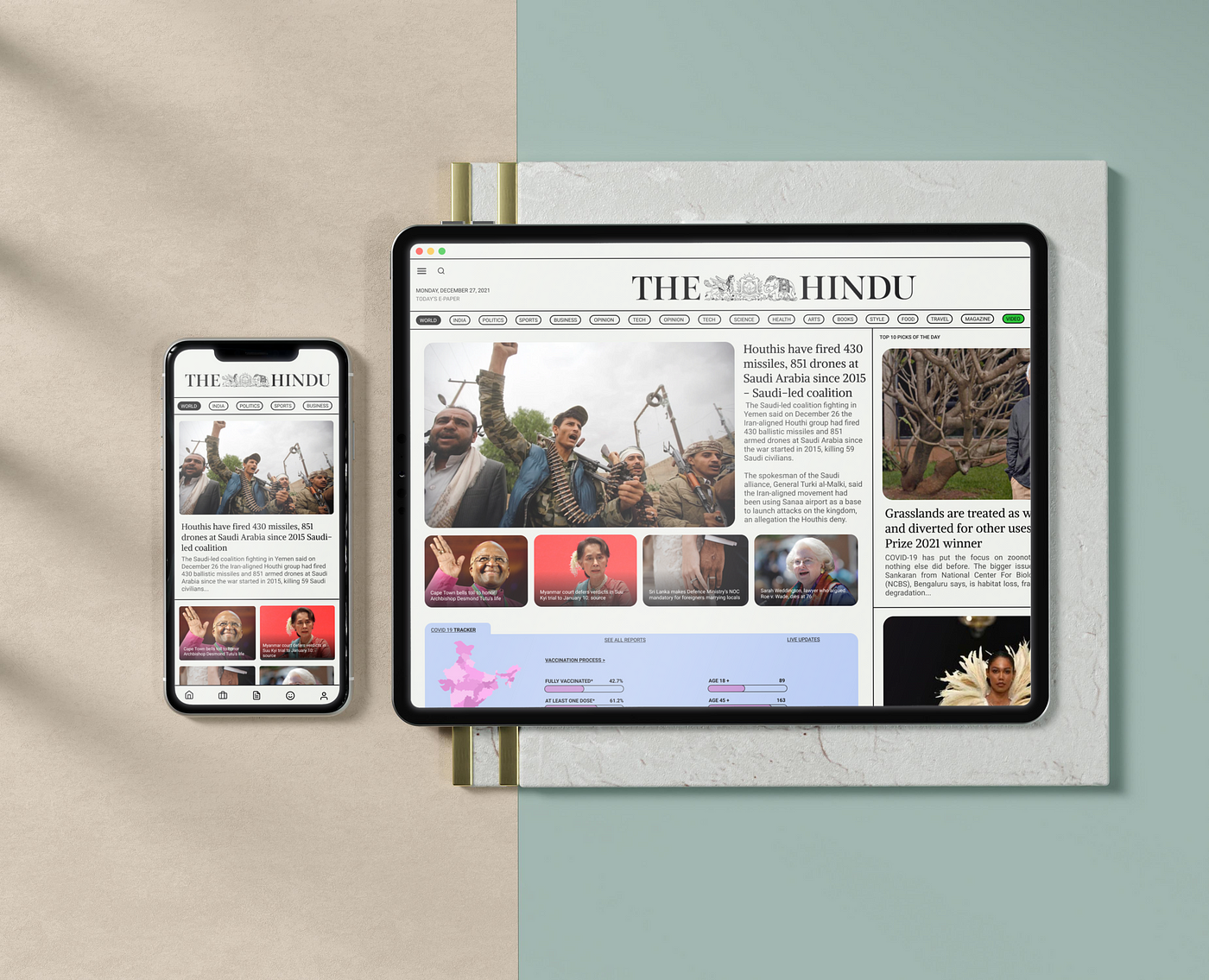The image showcases a black tablet and a black smartphone, positioned next to each other under cloths on what appears to be a bi-colored table. The left side of the table is light pink while the right side is light blue. The background wall is two-toned, with the left side in beige and the right in sage green, featuring a white square with two vertical gold stripes. Both devices are opened to the same front page of the online news website, The Hindu, displaying an article about the Houthis firing 430 missiles and 851 drones at Saudi Arabia since 2015. The webpage on both screens includes a prominent image of a man holding up his arm in triumph with artillery bullets around his neck, accompanied by other people. Below are multiple smaller, illegible images and captions, along with various news sections including public figures, grasslands, and fashion stories. The tablet rests on a light gray book with a gold metallic edge. The overall scene appears to combine real-life elements with digital editing for a vivid and detailed composition.